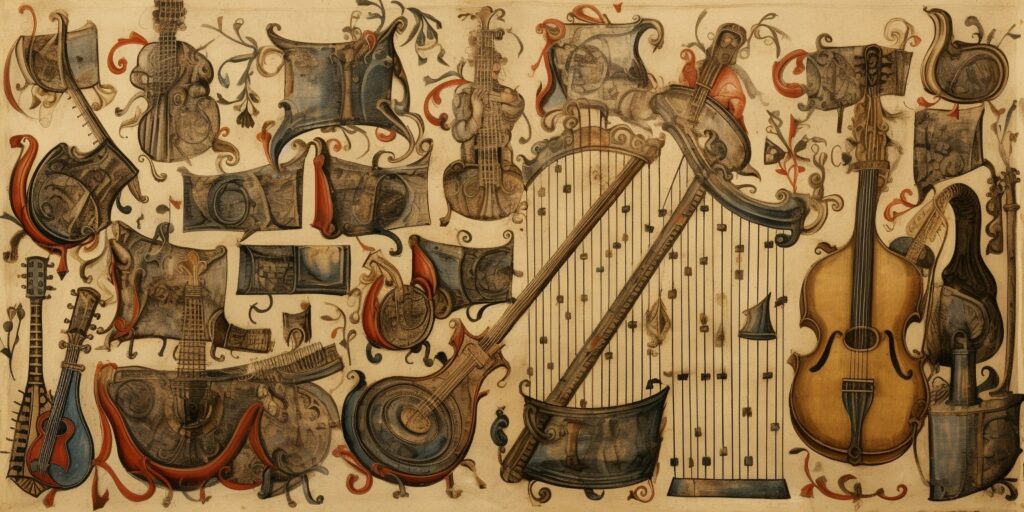This detailed drawing captures a medieval-inspired array of musical instruments against a light brown background, offering an elaborate and historical feel. On the left-hand side, a couple of small guitars are illustrated in the bottom corner. At the center, a man is depicted playing a cello, adding to the dynamic essence of the image. The right side features a large bass, prominently displayed. Various instruments in shades of brown, light brown, red, and blue are scattered and organized in rows across the image, contributing to the overall theme. Among them, a blue guitar with red accents near the strings stands out. Other notable instruments include dark brown mandolins, violins, a harp-like instrument with strings hanging down, and a large violin. Additionally, there are various brown objects, including a rolled-up item and a flag, enhancing the intricate composition of this medieval-styled artwork.